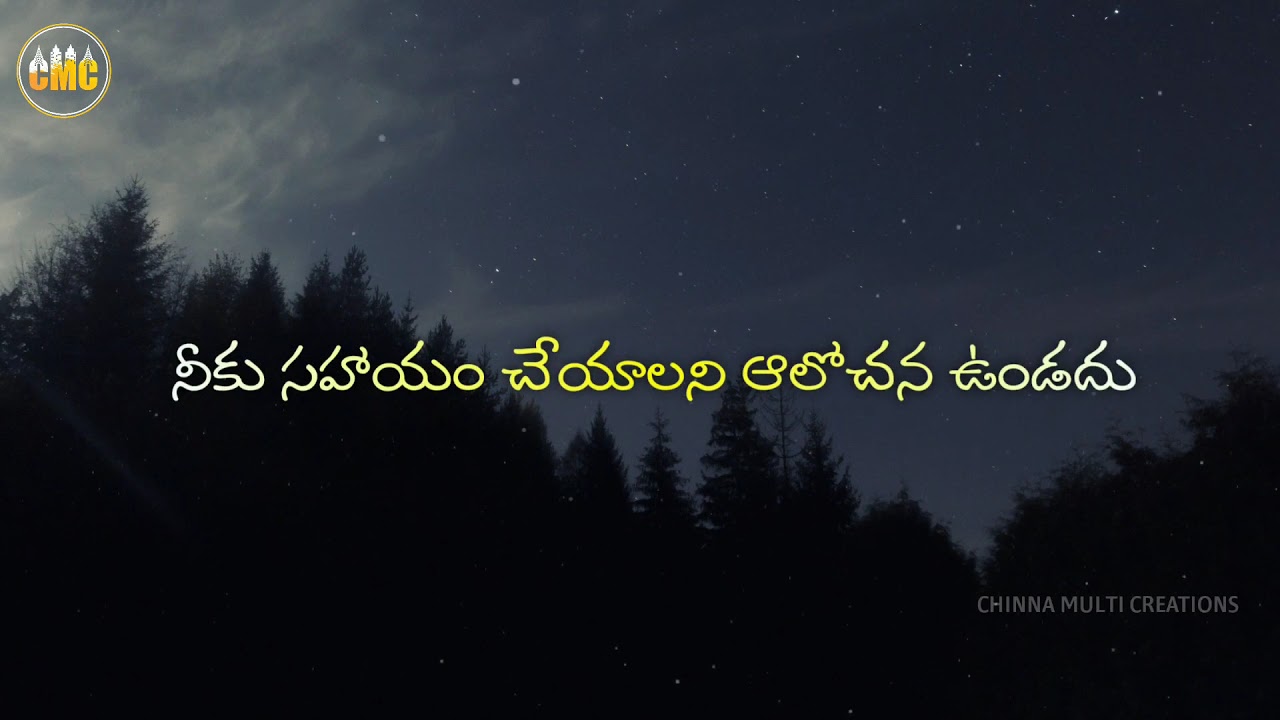The image is a nighttime photograph capturing an upward view of the sky and treetops. The night sky is a deep blue with scattered stars starting to reveal themselves. Wispy, partially transparent clouds drift in front of a subtle light source coming from the upper left corner. Silhouettes of evergreen trees are visible against the darkened sky. Across the center of the image, there is a line of foreign text in a script resembling elvish or possibly a form of Hindu, written in a yellow hue. In the lower right corner, there is a watermark consisting of a circular logo with an orange gradient font that reads "CMC," each letter adorned with a unique symbol. Below this, in white capital letters, the text reads "CHINA MULTI CREATIONS." The composition beautifully melds natural elements with textual overlays, creating a visually striking nocturnal scene.